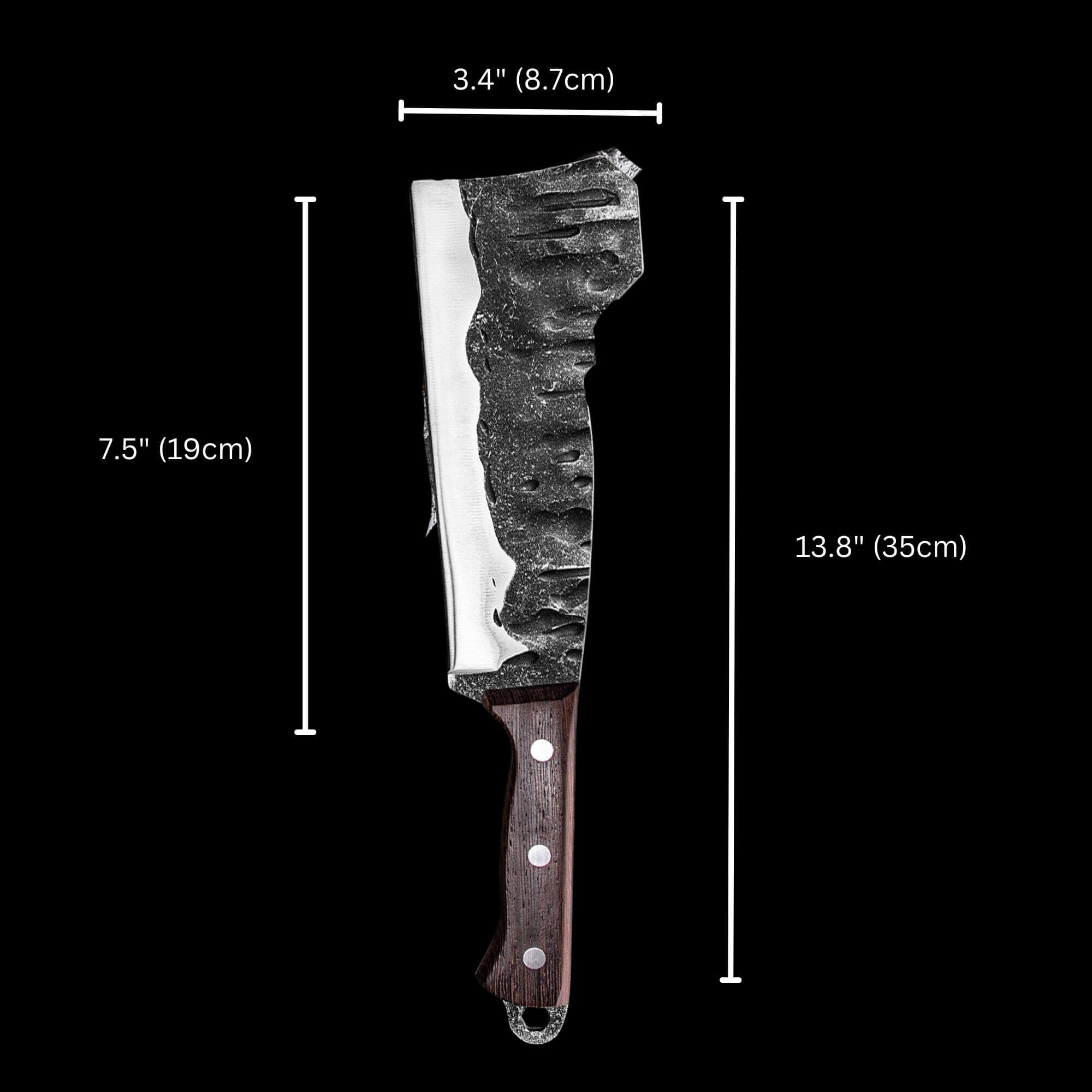This image features a large cutting knife prominently displayed against a solid black background. The knife has a thick, silver blade measuring 7.5 inches (19 centimeters) in length, and the overall length from the top of the blade to the bottom of the wooden handle is 13.8 inches (35 centimeters). The width of the blade is 3.4 inches. The dimensions are clearly shown in white text on the image. There are no additional graphics or text besides these numerical details.